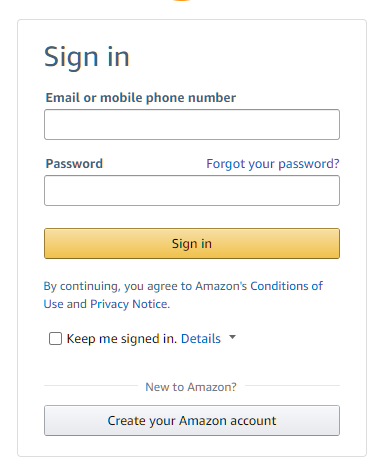**Caption:**

The image depicts the sign-in page for an Amazon account, framed by a very thin, black rectangular border. At the top left, the page starts with the word "Sign-In" in black text. Directly below, the label "Email or mobile phone number" appears in black, with a corresponding white rectangular input field beneath it for users to enter their information. Further down, there is the label "Password" next to another identical white rectangular field for entering the password. Adjacent to the password field, "Forgot your password?" is written in light blue text.

Furthermore, below the password input field, positioned to the right, is a rectangular yellow button containing the word "Sign-In" in black text. Following this button, a statement reads "By continuing, you agree to Amazon's Conditions of Use and Privacy Notice." Below this statement, there's a checkbox option labeled "Keep me signed in. Details." At the very bottom of the image, a final section reads "Create your Amazon account," providing an option for new users to register.